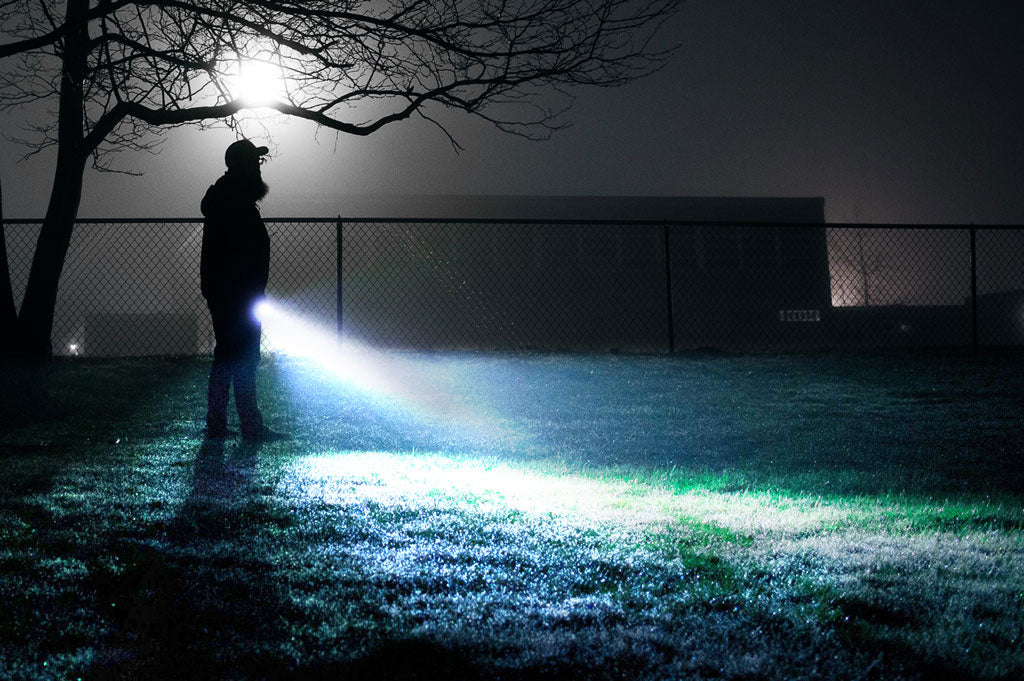In this black and white nighttime photograph, a medium-built man, likely a security guard, is seen in silhouette, facing right. He wears a baseball cap, possibly glasses, and a jacket, suggesting a cold environment. The distinct beard highlights his male identity. He holds a flashlight in his right hand, casting light onto a green lawn with hints of blue shades, indicating humid grass. Behind him stretches a chain-link fence with a barren tree and an indistinct building displaying a numbered sign. The sky is predominantly dark, lit only by a bright moon hanging directly above his head, lending a silvery hue to the scene. The image captures a solitary, late-night moment, devoid of other people, animals, or vehicles.